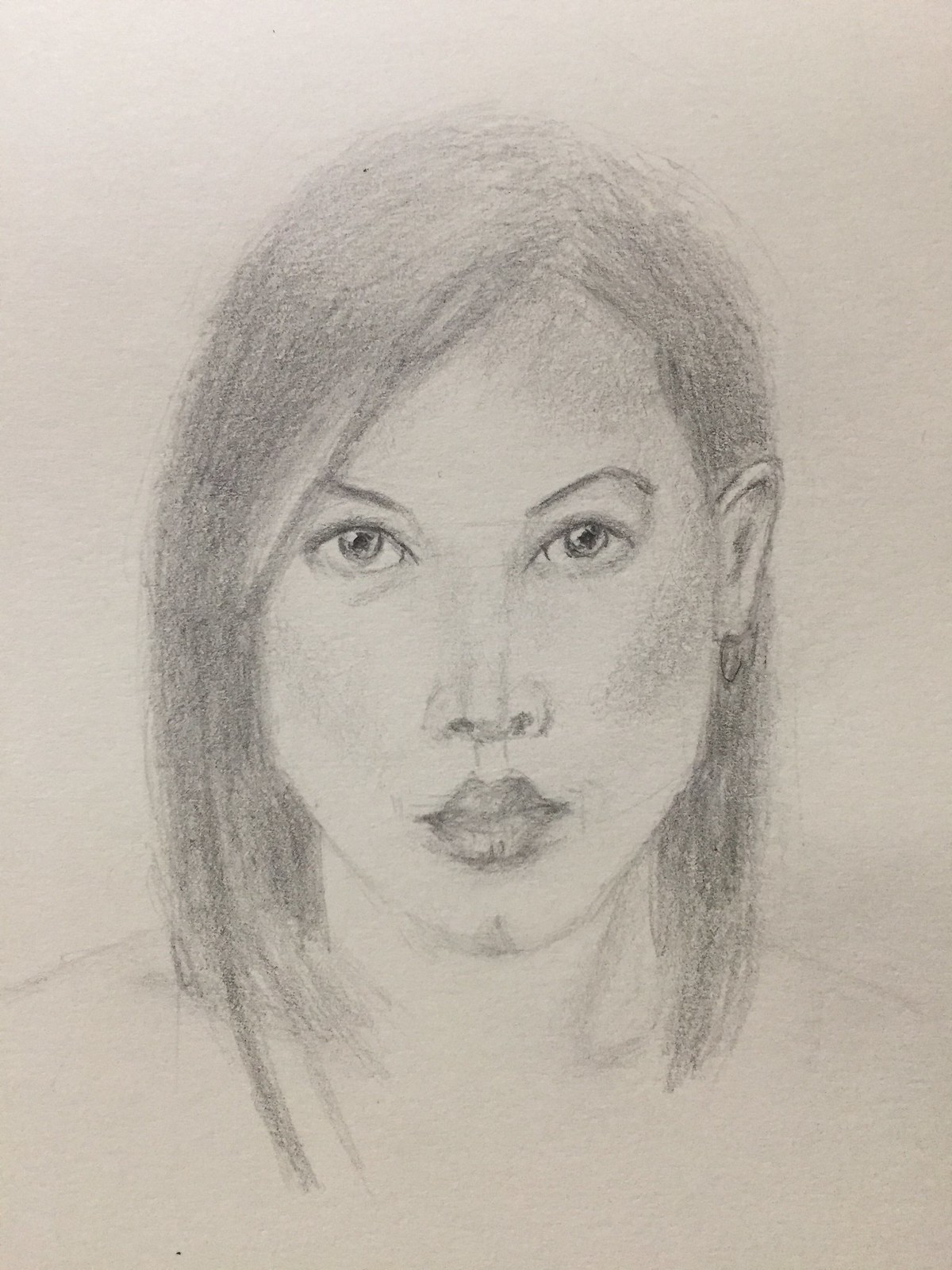This image is a detailed pencil sketch on an off-white sheet of paper, depicting a woman from her head down to her shoulders. She is looking straight forward. Her straight, shoulder-length hair has a side part; it slightly covers her left eye and is tucked behind her right ear, revealing a hoop earring. She has thin eyebrows and oval-shaped, slightly baggy eyes with prominently dark pupils that have a luminous quality. Her nose is round with upturned nostrils, and there are slight lines extending from the base of her nose to her lips. Her lips, which appear squished or pursed together with a slightly triangular shape on top, rest above a subtle chin dimple. The shading around her neck softly outlines her form, while the fine shadowing on her cheeks accentuates her delicate, oval face and slightly strong jawline or "butt chin."